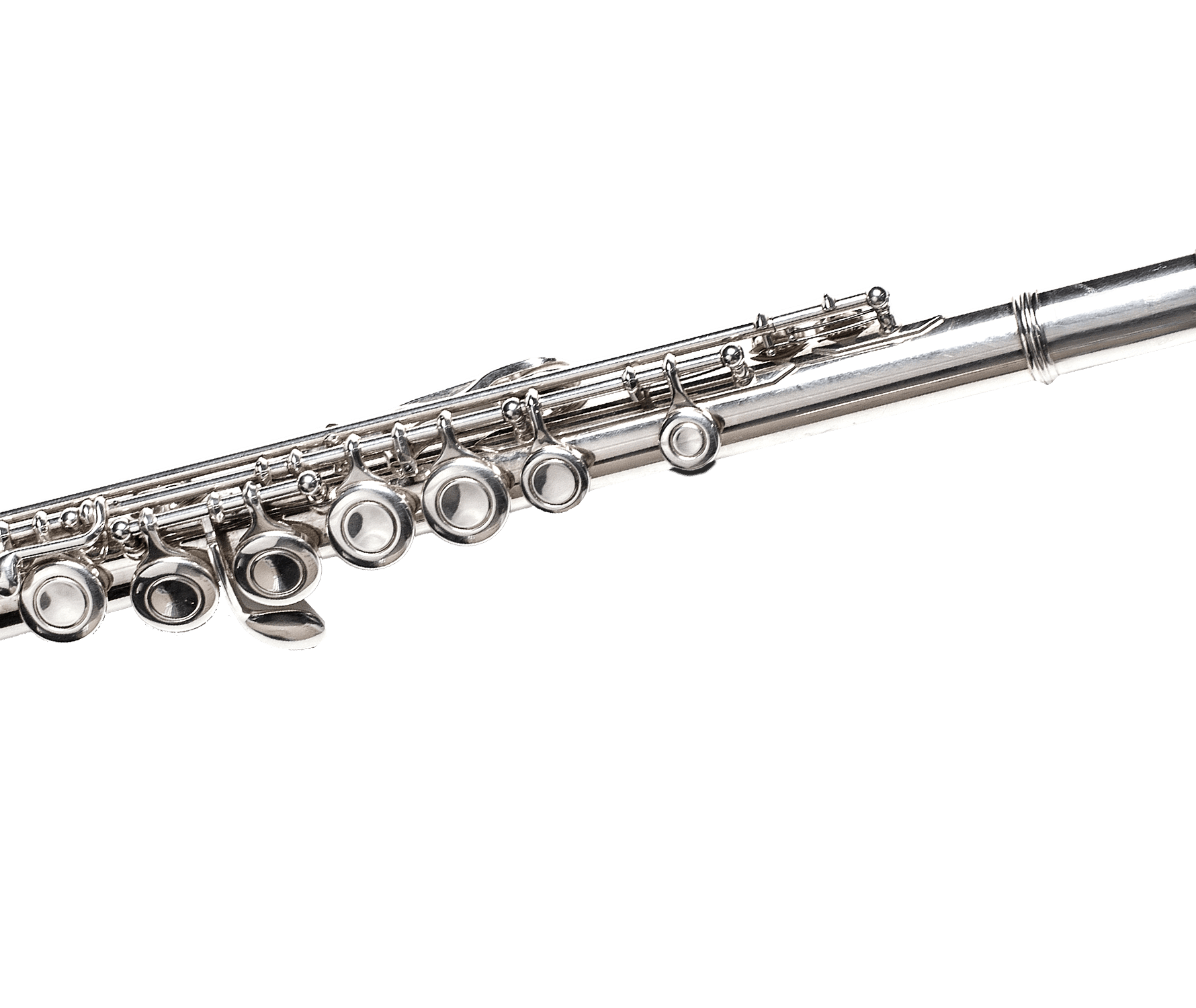The image features a close-up view of a silver flute set against a white background, possibly the screen of a computer laptop. The flute is slanted so that the wider part is towards the left-middle of the image, while the narrower end points just above the right-middle. The flute's buttons, predominantly on the left side of the picture, catch the light and shine in varying shades of silver, gray, and black. There are seven round buttons visible, connected by three intricate bars. The right end of the flute is simpler, showcasing the smooth, ringed barrel leading towards the mouthpiece. Despite the detailed view, there is no shadow cast on the background, making the flute stand out prominently.